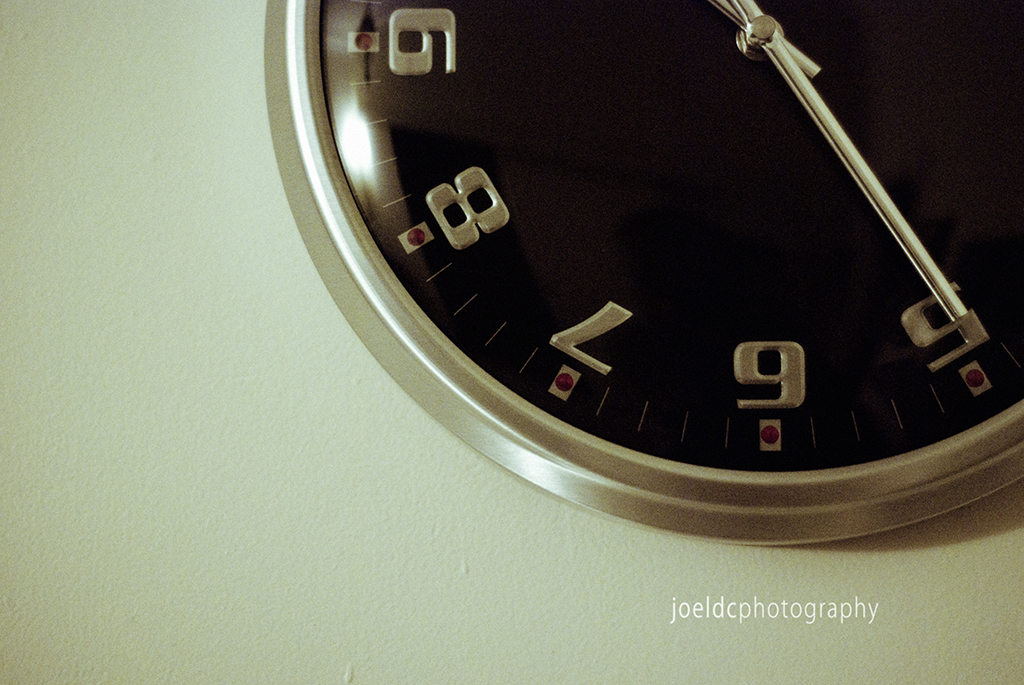The image displays the lower left quarter of a dark chocolate brown clock face, prominently showing the time from 5 p.m. to 9 p.m. The minute hand, a whitish silver in color, is fixed on the 5. The rest of the dial is partially cropped out in the upper right corner, creating a focused view of the bottom left segment. The outer framing of the clock appears to be made of silver, enhancing its sleek and modern aesthetic. A greenish-tan colored wall serves as the background, providing a muted backdrop that contrasts with the clock's darker tones. In the bottom right corner, just beneath the clock's edge, the signature "Joel C. Photography" is elegantly inscribed in white lettering, adding a personal touch to the composition.